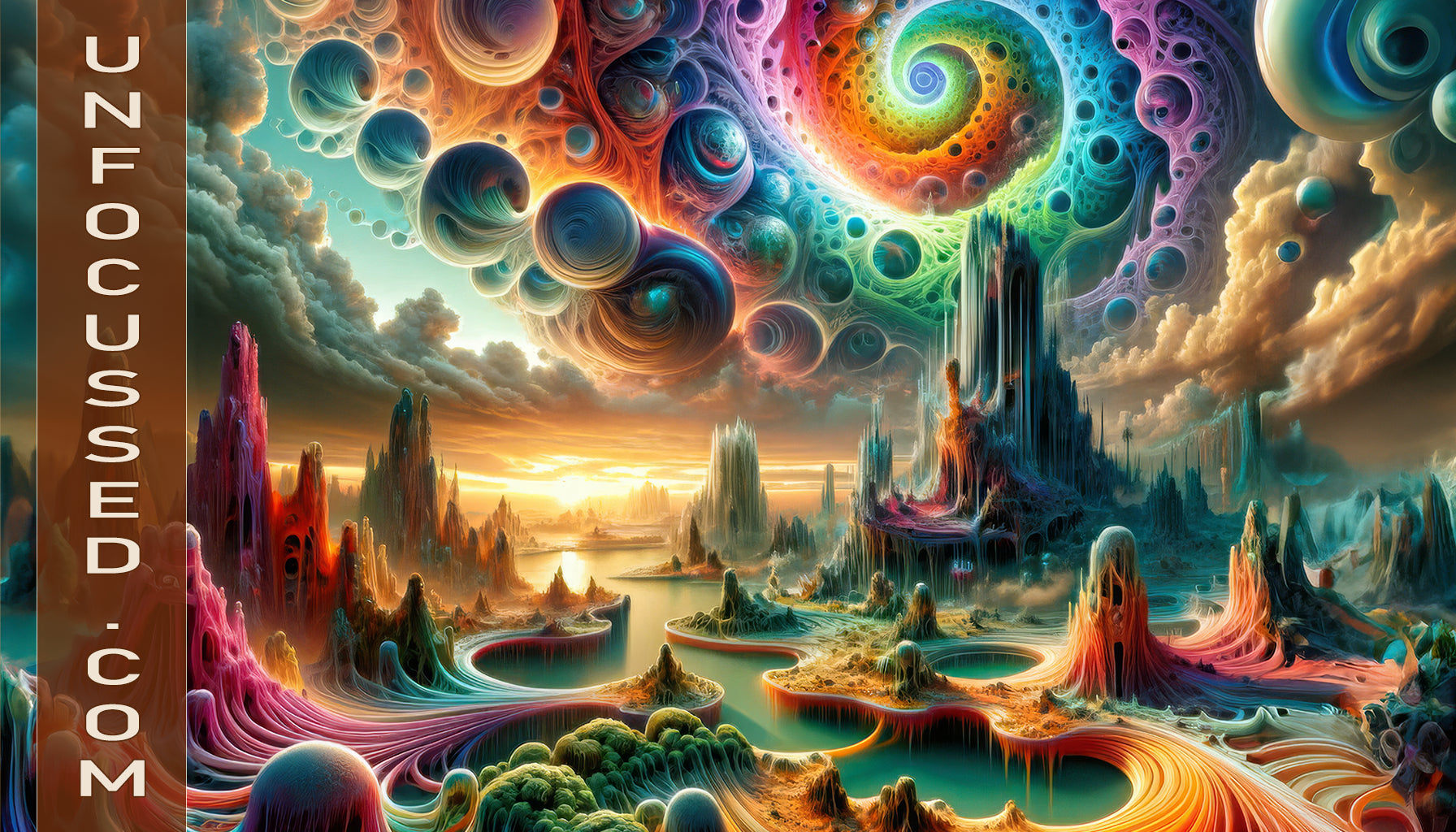The image is a digitally synthesized, abstract mythical outdoor scene, featuring a vibrant and fantastical landscape. This landscape is populated with tall, tower-like structures that resemble mountainous buildings, composed of swirling lines and a plethora of vivid colors including green, blue, orange, pink, and red. A river of green, aqua-blue water winds through the middle of the scene, accentuating the colorful land formations on either side. To the right of the center, the tallest structure stands prominently, rendered in a dark blue shade, with another shorter, orange-colored feature in front of it.

Above the scene, the sky is adorned with a swirling abstract pattern, boasting a rainbow of colors that coalesce into circular swirls, resembling an octopus leg, rising above clouds with golden and light blue tones. This swirling pattern is most prominent above the tallest blue structure. On the left side of the image, there's a significant vertical banner stretching from the top to the bottom. It is brown and semi-transparent, with the text "unfocused.com" written in white letters stacked vertically from top to bottom.

Further details include bubble-like formations around the central areas of the image, some appearing dark and hole-like, while others look like clear air bubbles. The surrounding swirls feature layers of pinks, purples, blues, and oranges, with green protrusions within some swirls. This imaginative world below the abstract sky consists of jagged and pointy elements resembling stalactites and stalagmites, with curved and flat shapes interwoven, suggesting an otherworldly landform beneath an exotic, swirling canopy.